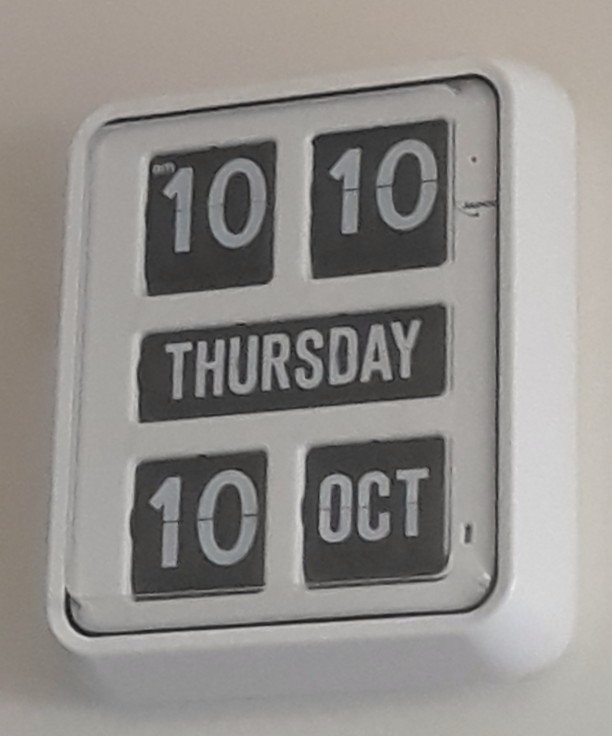A light gray wall serves as the background for a square, white plastic clock with rounded corners. The clock face is also white and features two black square windows at the top, displaying the white numbers "10:10." Below these, a black rectangular box indicates the day of the week, reading "Thursday" in white letters. Further down, two additional black square windows showcase the date, with "10" and "October" clearly marked in white. The clock exhibits some scratches on its side, and there is a small hole near the bottom, close to where the month is displayed.